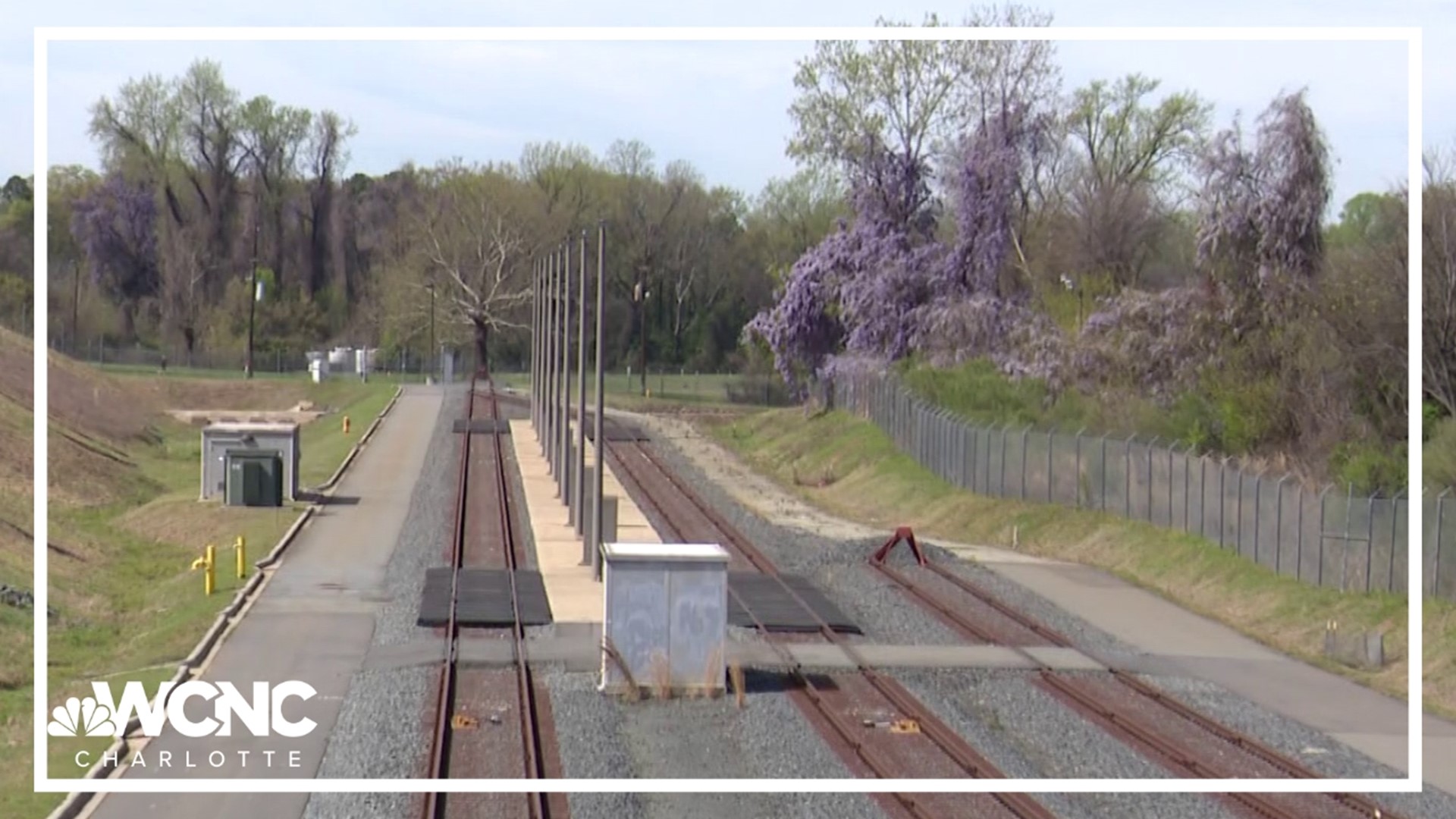The image depicts a serene outdoor train station with three distinct railway tracks. The tracks, which are a rusty brown color, include two that extend into the distance and curve, and one shorter track on the right that terminates visibly. Between the tracks, there are several sturdy gray metal poles, likely supporting electrical lines or signage. The area surrounding the railways is lush with greenery, complemented by patches of green grass on both the left and right sides. In the background, a mix of green trees and some striking pinkish-purple trees with vibrant flowers adds a touch of vibrant color to the scene. On the far right side of the image, a wide gray fence runs parallel to the tracks. An electrical box is also visible near the fence. At the very bottom left of the picture, the text "WCNC Charlotte" suggests that the image might be from a news feed or associated with a news station.